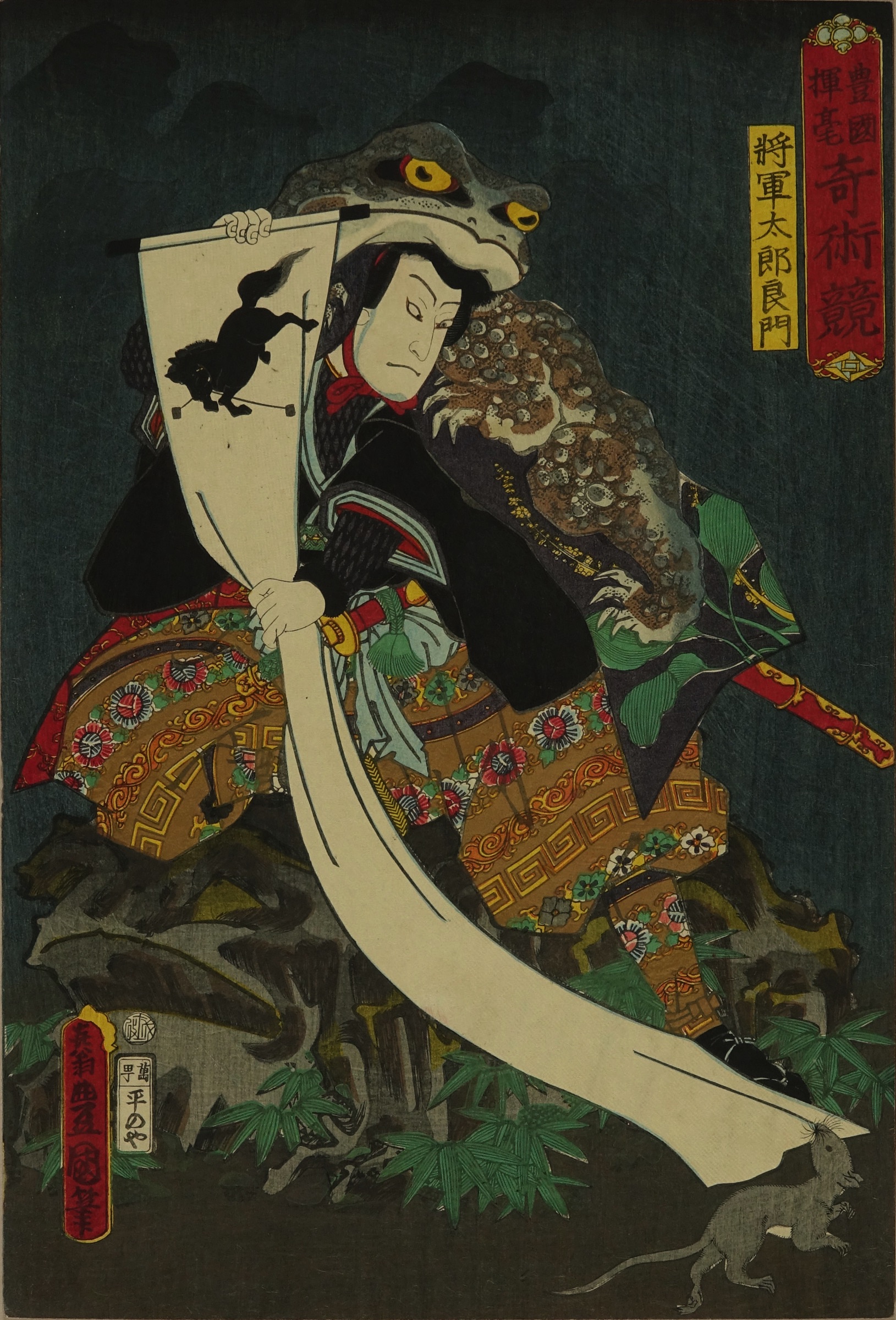The image is a rectangular, classic Japanese painting approximately six inches high and three to four inches wide. It depicts an Asian man with his face painted white, characterized by a frown, thin black eyebrows, and upturned slanted eyes, gazing downward toward the lower right-hand corner. The man wears a black long-sleeve top and colorful brown, fluffy pants. Resting on his head and back is a large gray and brown toad with vivid yellow eyes. The background transitions from dark grays at the top and center, imitating the ground with brown hues at the bottom.

In his arms, the man holds a long white scroll that features the image of a black horse in motion. A gray mouse is tugging at the end of this scroll in the bottom right-hand corner. Surrounding the central figure are various pieces of Japanese writing: a small vertical golden rectangle with black script in the upper right-hand corner, a large red oval with black lettering to the left, and another vertical red oval in the lower left-hand corner, with additional black characters on a white rectangle to the right of it. Overall, the intricate details and traditional attire convey the essence of an ancient Japanese artwork.